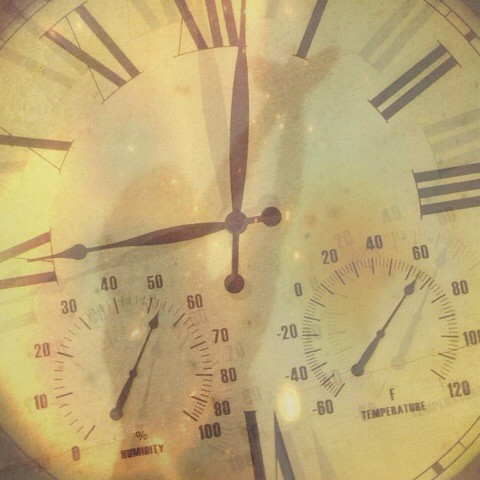A detailed close-up composite of a clock face reveals a dim reflection or shadow of a person in the center, their arms raised, creating a bird hand shadow with both hands crossed. The clock face features Roman numerals, partially visible around the edges, with the time indicating a few minutes past 9 o'clock. Smaller dials are integrated into the clock face: one shows the Fahrenheit temperature as 63 degrees, while another on the left side displays the humidity at 52%. The photograph's composition highlights the intricate interplay of shadows and reflections, lending a mysterious and intricate quality to the image.